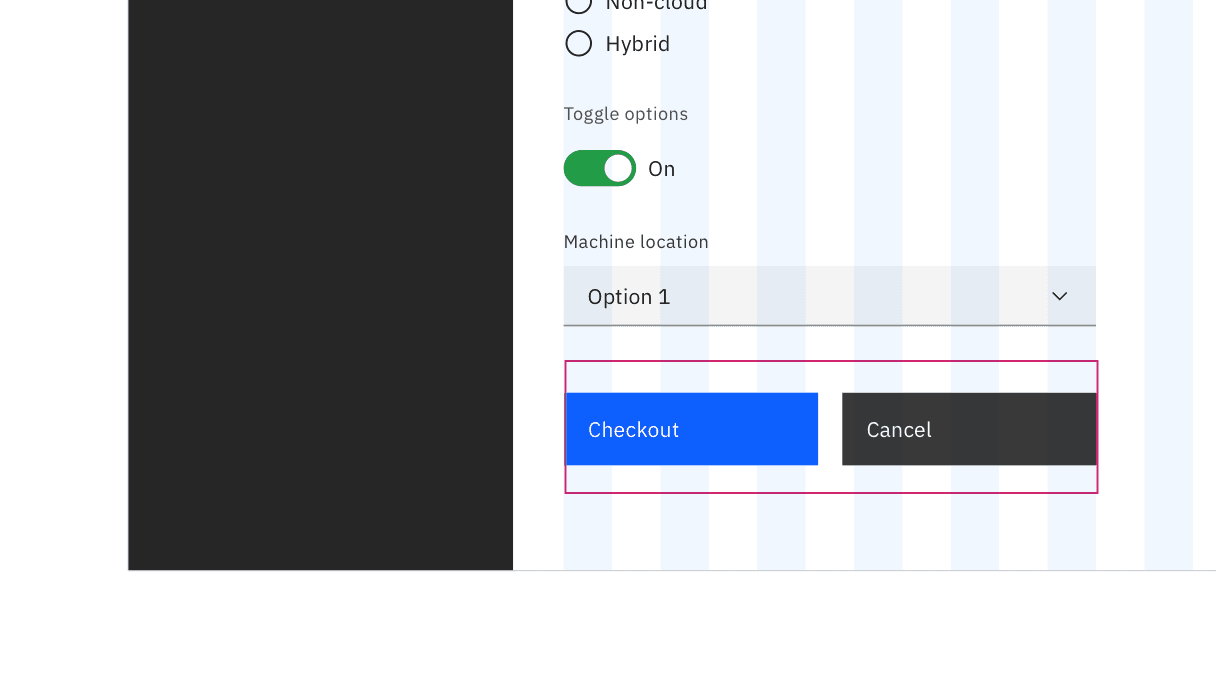In this image, we see a cell phone in landscape orientation. The left third of the screen is entirely black, suggesting that only part of the phone's screen is captured. The remaining two-thirds of the screen display a user interface. At the top, there are partially visible words, suggesting that the content has been scrolled to the bottom. Prominently displayed is the word "Hybrid" accompanied by a toggle button, which appears to be activated. Below this, there are the words "Toggle Options" followed by another active status indicator. Further down is an entry labeled "Machine Location" with a drop-down menu set to "Option 1". 

At the bottom of the interface, there are two large rectangular buttons. The first is blue and labeled "Check Out," while the second is black and labeled "Cancel." The background of this settings screen features a pattern of vertical stripes in alternating colors of white and light blue, adding a subtle visual texture behind the interface elements. The overall composition suggests a settings or configuration screen for a machine or application, captured in a moment of user interaction.